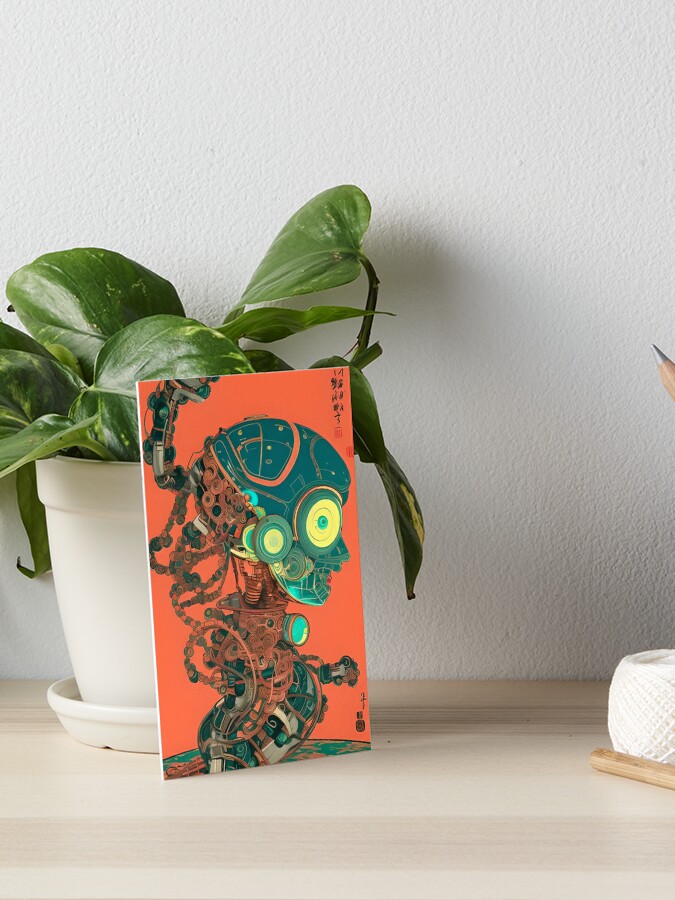The image features a light beige tabletop adorned with a small but lush green potted plant. The plant, housed in a white pot with a matching dish below, has broad, pointed leaves, though the thick stems are somewhat hidden. Positioned in front of the pot is a striking, abstract artwork piece. The artwork presents a mechanical figure with a dark blue, skull-like head that has a large, prominent yellow eye. The background of this piece is a vivid orange, accentuating the bold features of the robot-like figure. To the right of the plant and artwork, there's a spool of white yarn and a silver pencil tip visible on the table. The scene is set against a smooth, white wall, providing a clean and uncluttered background.